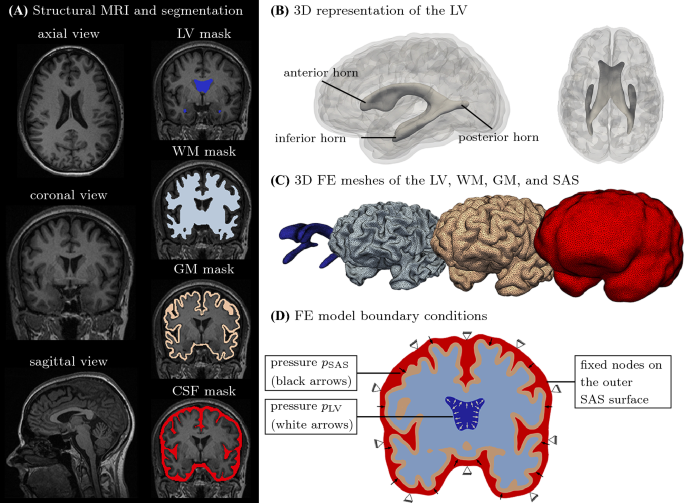This image showcases multiple detailed diagrams of the human brain, emphasizing structural MRI and segmentation views on a black-background frame. The top section, denoted as "A," presents three anatomical brain images, with axial, coronal, and sagittal views aligned from top to bottom. Adjacent to these, additional images illustrate LV, WM, GM, and CSF masks.

The midsection, labeled "B," features a 3D representation of the lateral ventricles (LV), highlighting the anterior, inferior, and posterior horns of the brain with specific pointers. The top right of this section includes a top-down view of the brain without annotations.

In the lower part, identified as "C," there are three distinct 3D finite element (FE) meshes colored blue, tan, and red representing the LV, WM, GM, and SAS, with an additional non-brain blue object.

At the bottom, denoted as "D," the FE model boundary conditions are depicted, showcasing a brain image with a blue interior and a red border. This section includes pressure annotations: PSAS with black arrows and PLV with white arrows, alongside fixed nodes on the outer SAS surface highlighted in black font.

In summary, this composite image uses a primary color palette of gray, beige, red, and shades of blue to present extensive, multi-angled, and segmented representations of the human brain.